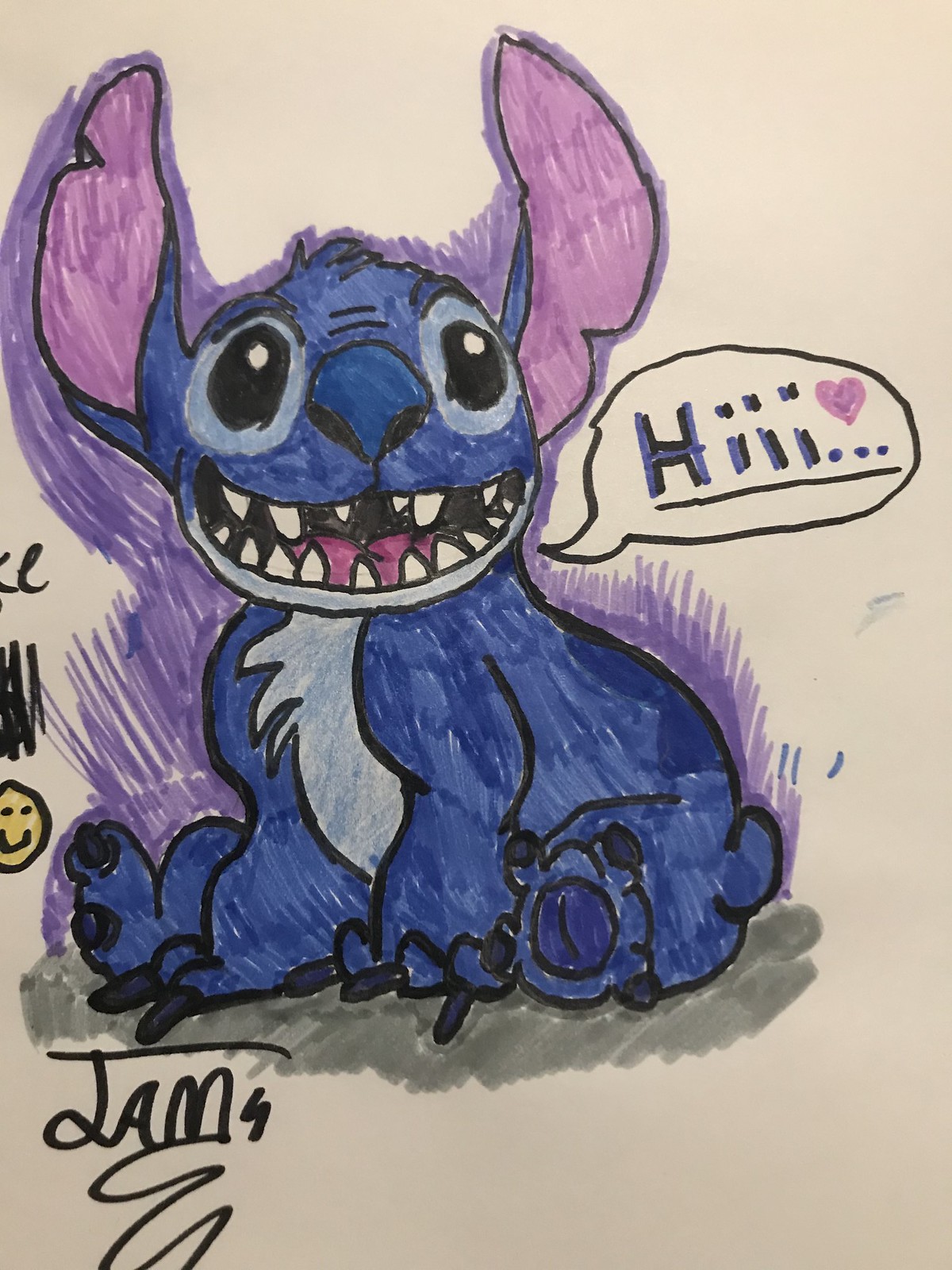This vibrant drawing, created with marker, vividly depicts a whimsical koala bear with unconventional features. The bear, predominantly blue in color, boasts large ears that extend sideways before curving upwards, with the inner portions painted pink. The creature's sizeable, expressive eyes and roundish nose immediately draw attention. Parting its mouth wide open, the bear reveals an array of sporadic, sharp teeth. Its chest stands out in stark white contrast to its blue body. Adding a touch of communicative charm, a speech bubble emerges from the right side of the bear’s mouth, greeting viewers with a cheerful "Hi."